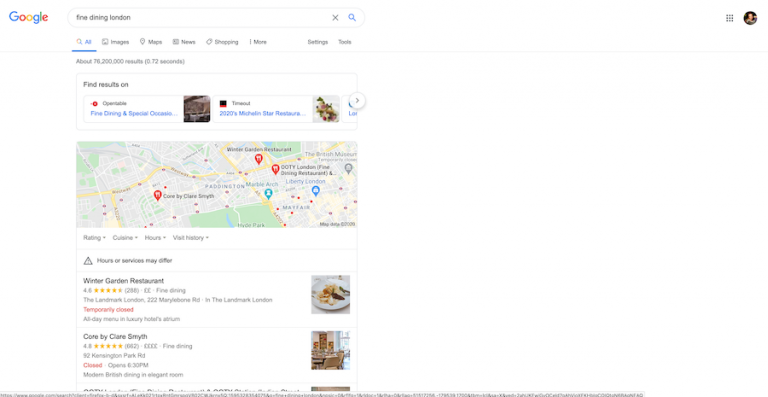This screenshot captures the Google search results page for the inquiry "Fine Dining London." Displayed on a clean, white background, the Google search bar is prominently featured at the top center with the query text entered. Directly below the search bar is a horizontal menu featuring options like All, Images, Maps, News, Shopping, and More, with "All" highlighted in blue, indicating the general search results are currently being viewed.

The search results reveal there are approximately 76 million entries, retrieved in just 0.72 seconds. Located further down the page, a dynamic map of London highlights several fine dining establishments. Noteworthy among the top search results are the Winter Garden Restaurant and Core by Clare Smyth, each accompanied by their Google review ratings, cost information, location, and operating hours.

The detailed entries for these restaurants provide valuable insights, including the ability to click through for more information, explore their menus, and read reviews from other patrons. This arrangement offers a comprehensive starting point for anyone looking to explore the fine dining scene in London.